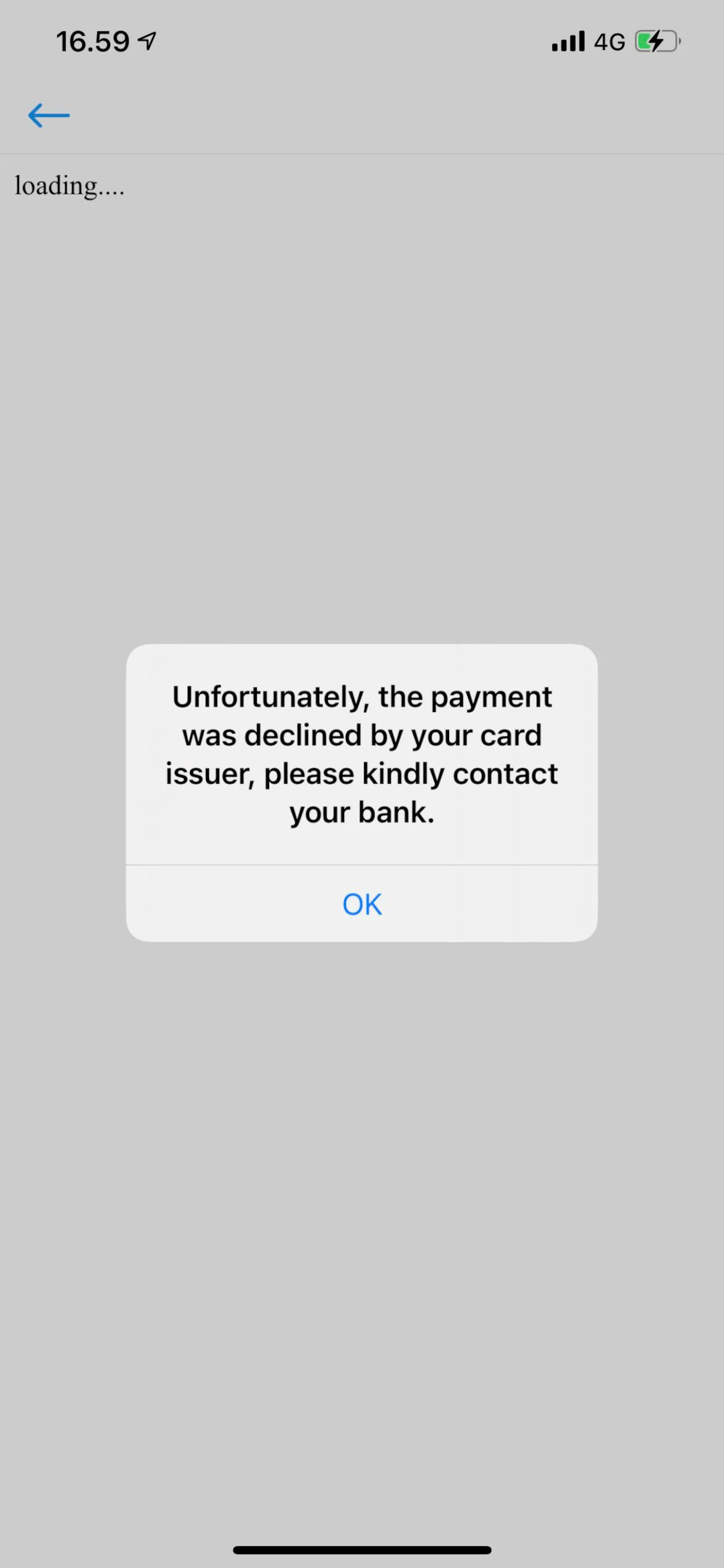The image is a screenshot captured from a smartphone. The phone itself is not visible, only its screen is presented. The top left corner displays the time in military format as "16:59," accompanied by an upward-pointing arrow. Adjacent to this on the top right corner are four fully lit signal bars indicating maximum connectivity, and a "4G" label signifying 4G network coverage. Next to these indicators is a battery icon, distinguished by a lightning bolt symbol within it, suggesting the battery is currently charging.

Below the status bar, the left side of the screen features a blue arrow icon above a thin horizontal line. This line appears to animate a loading process with four pulsating dots beside it, indicative of an ongoing action or data being processed.

The central part of the screen displays a notification, housed in a white square with rounded edges. The message reads: "Unfortunately, the payment was declined by your card issuer. Please kindly contact your bank." Beneath this text, a separator line is visible, with the word "OK" in blue font positioned below it, suggesting an action button for dismissing the message.

At the very bottom of the screen, a thin horizontal line spans the center, possibly serving as a navigation or gesture indicator. The entire background of the screen is a solid grey color, with sharp square borders defining the edges.